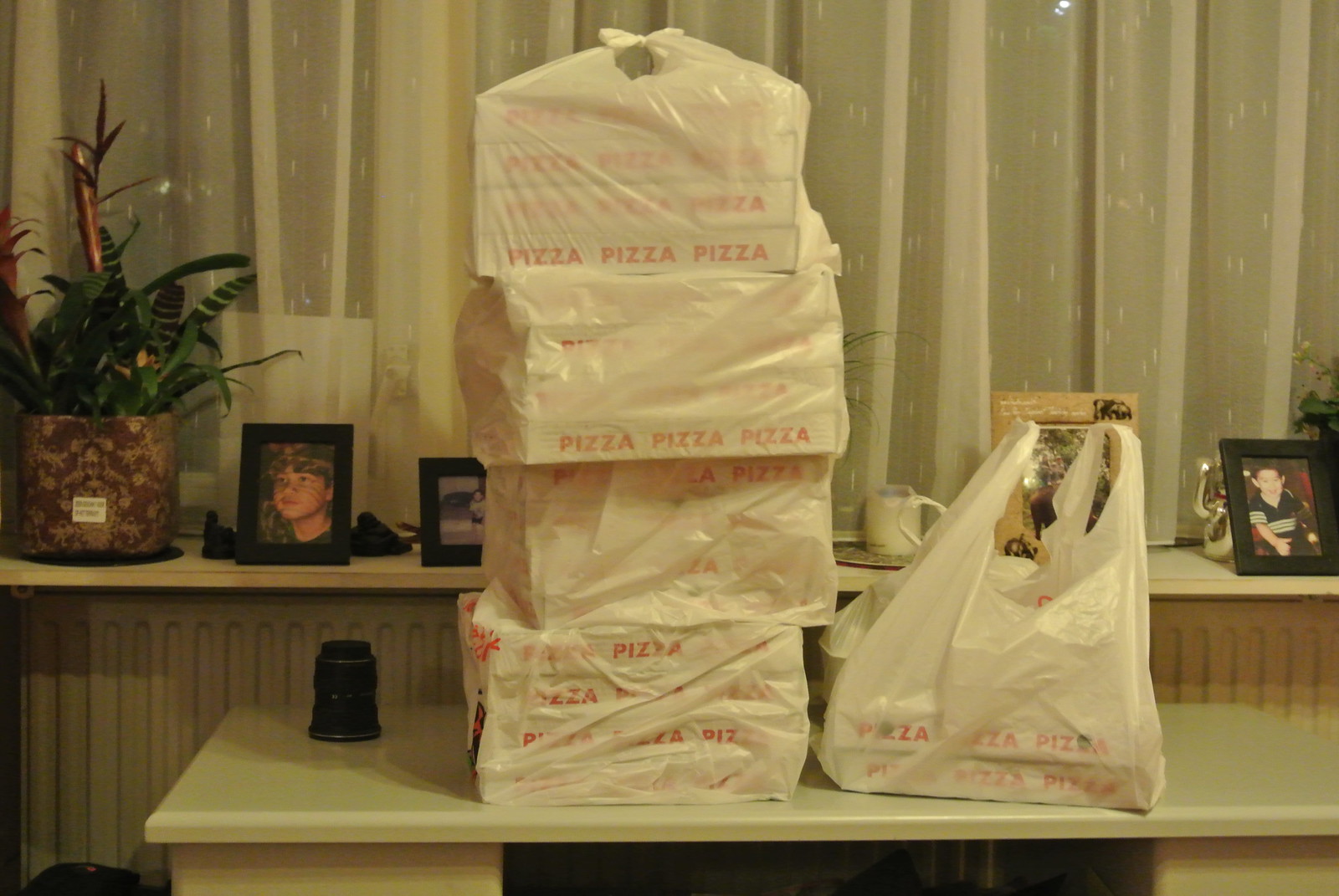This indoor photograph captures a cozy living or sitting room, warmly lit by yellowish, typical indoor lighting. The focal point is a white desk in the foreground, topped with multiple white plastic bags containing pizza boxes. There are four bags, each holding four white pizza boxes, and a fifth bag containing two more boxes. Each box is labeled with "pizza pizza pizza" in red text.

Behind the desk, a window is adorned with net and white satin curtains, partially revealing the dark outside. Below the window, a shelf or ledge holds several black-framed family photos and a vibrant green plant in a brown-and-tan styled pot. Additionally, there is a black cylindrical cup positioned at the back left corner of the desk. The scene radiates a homely and intimate ambiance, with the pizza delivery adding a casual, lived-in touch.